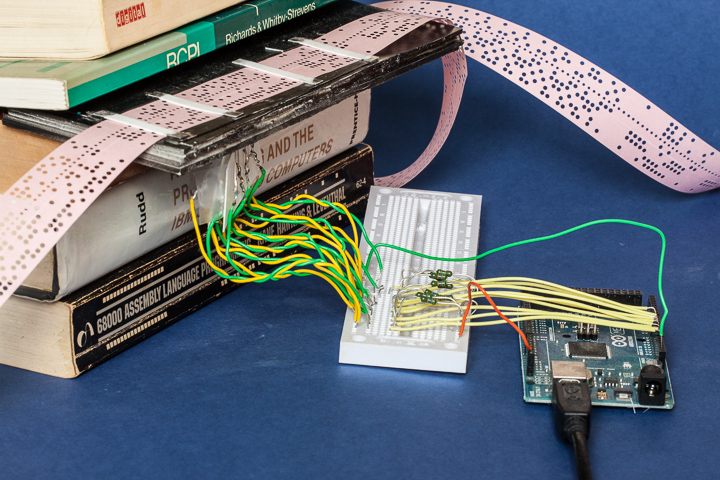This detailed photograph showcases a cluttered stack of five books, set against a dark blue flat-colored table. At the heart of this scene is an array of electrical components that evoke a sense of computer technology. On the third book from the bottom, a pinkish plastic ribbon connector sits prominently, resembling the type used to attach hard drives. This ribbon connector is punctuated with numerous dots and is flanked by a bundle of green and yellow wires. These wires run intricately into a white rectangular encasement, from which more yellow wires and a solitary green wire extend towards a green circuit board adorned with black microchips and components. A USB connector is visible on the left side of this circuit board, further emphasizing the technological theme. The meticulous arrangement of these elements against the untidy stack of books creates a strikingly detailed and layered scene.